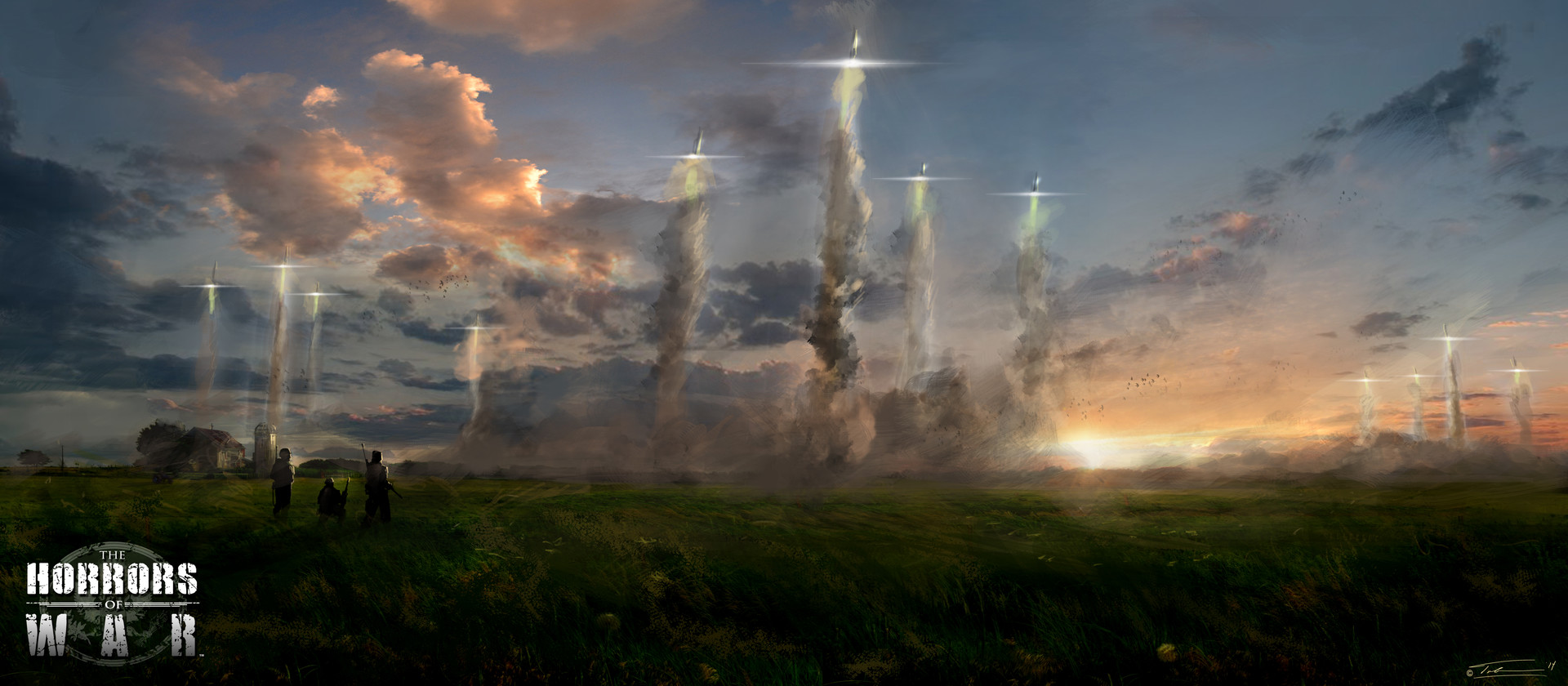The painting, likely an oil piece, titled "The Horrors of War" (text displayed in white, stencil-type font on the bottom left, through a modern watermark), captures a panoramic view of a once beautiful countryside now marred by war. In the foreground, a vast green field stretches out, with three figures standing on the left, their backs turned as they witness the devastation. In the background, a small farmhouse sits, seemingly untouched. The sky, transitioning from light blue to a foreboding dark gray as it fills with billowing clouds, further sets the somber mood. Dominating the scene are numerous bomber aircraft, a total of twelve, with eight on the left and four more in the distant background, releasing dark smoke trails as they rain destruction upon the land below. The sun hovers low on the horizon, casting its fading light and enhancing the drama of the scene.